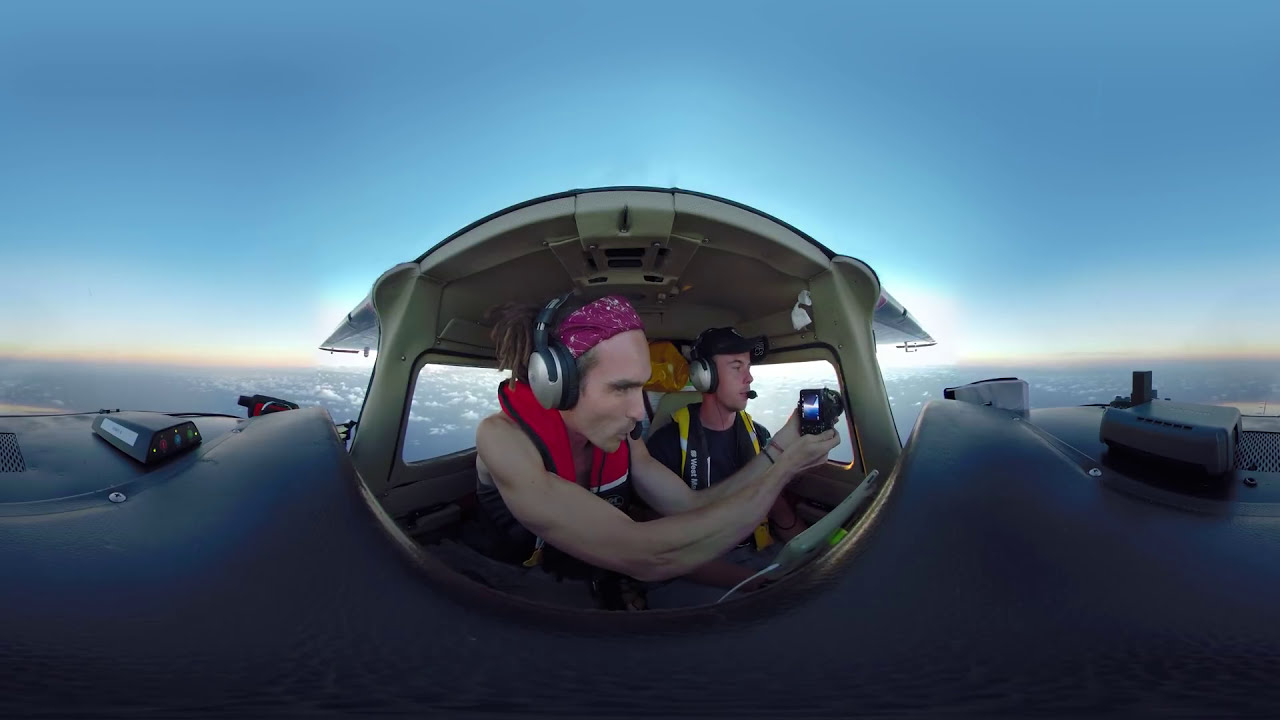The image is a vibrant 360-degree view inside a plane, capturing two men in a cockpit, flying above the clouds under a bright blue sky. The man on the left sports a pink bandana over his dreadlocked hair, secured in a ponytail, and he wears large silver headphones paired with a red safety vest over a black tank top. He is intently holding a camera out of the window, looking to the right. Beside him, the other man dons a black baseball cap, silver headphones, a black shirt, and a black and yellow strapped backpack. Both are gazing out of the window to the right, with microphones from their headsets positioned in front of their mouths. The cockpit, made of a tan plastic material, extends to the left and right as indicated by the 360-degree perspective. There is a screen with a plug visible in front of them, likely part of the plane's instrumentation. The foreground includes the wing and part of the plane's side frame, set against a backdrop of expansive clouds and a wide open sky that amplifies the sense of flight.